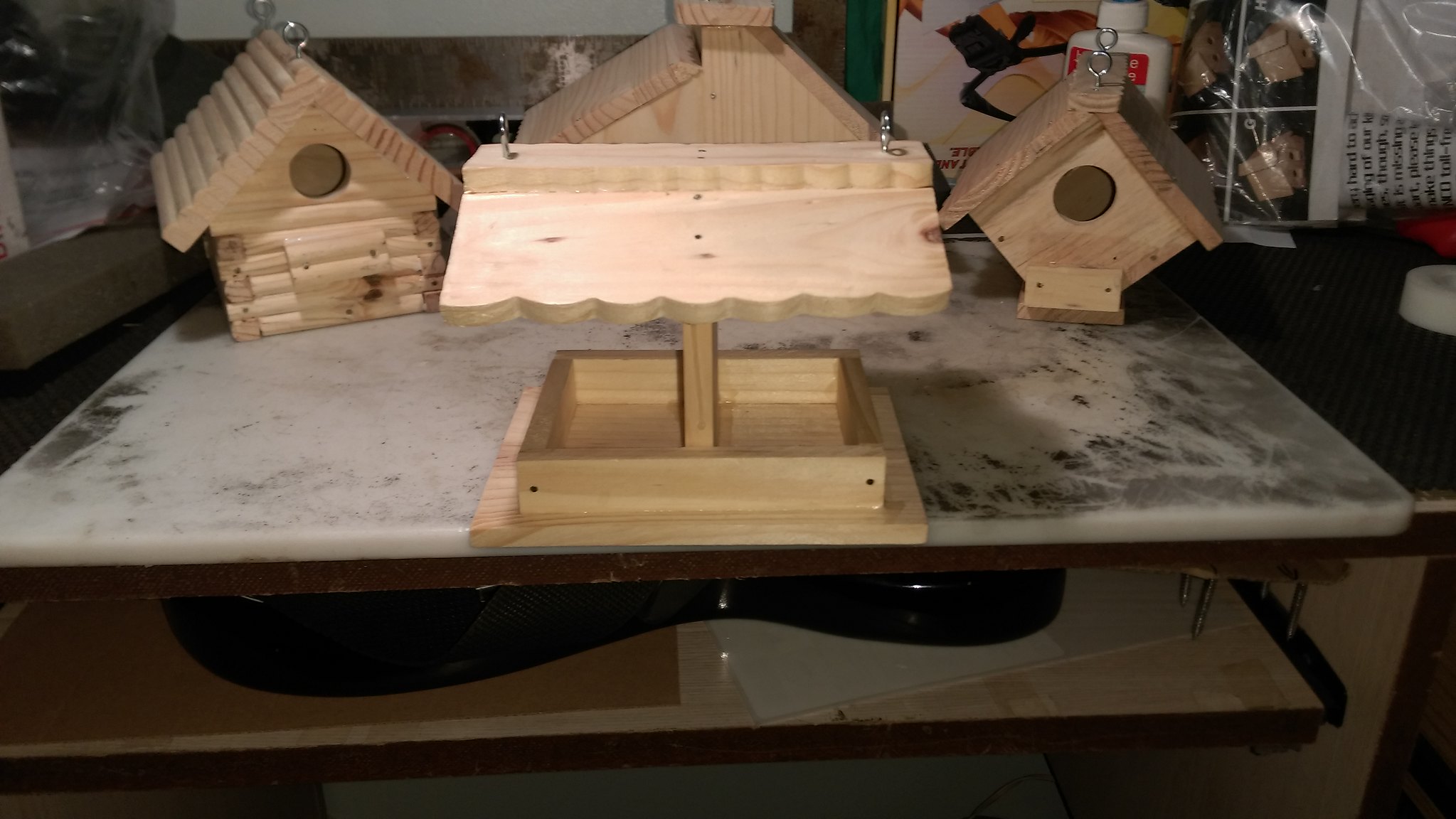The image captures an amateur photograph taken in a dimly lit wood shop or garage, showcasing a close-up of newly constructed wooden birdhouses on a well-used work table. The birdhouses, still in their raw, unstained wood form, display different styles. On the left, a log cabin-style birdhouse with a textured surface and arched roof has a small entry hole at the top. In the middle, a birdhouse resembling a feeder features hooks on top and an integrated birdseed platform beneath its arched overhang. The rightmost birdhouse, diamond-shaped with an arched roof, is accompanied by a partially constructed house next to it, comprising only a base, central support, and a small roof. The white work table, marked by stains, dirt, and gray smudges, reflects years of use and contains a shelf underneath holding black items. Behind the birdhouses, various craft supplies, including a bottle of glue and a soft-shell plastic container, are visible, along with some posters on the wall.